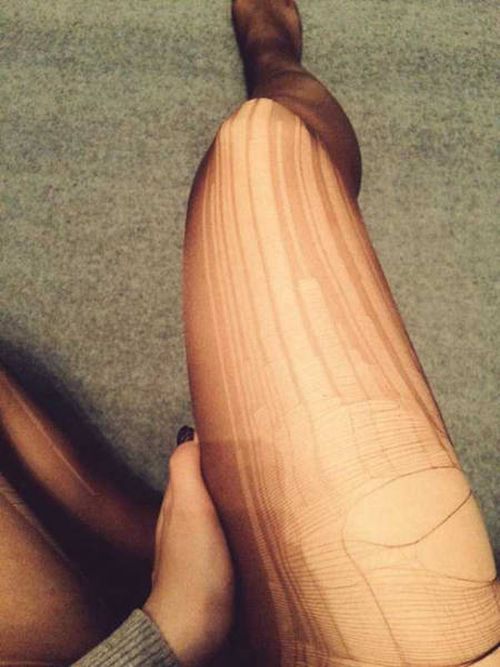In the image, a woman is sitting on a gray surface, either cement or carpet, with her legs prominently displayed. She is wearing a pair of badly run and torn dark nylon pantyhose. Her right leg is extended in front of her, completely riddled with runs and holes, especially pronounced around the thigh where two large holes are visible. Her left leg is bent beneath her, its foot tucked under the extended right leg, sporting fewer runs than the right. Her hand, adorned with dark purple nail polish on the thumb, supports her right thigh, and a gray long-sleeved sweater encases her arm. The image seems to portray a candid moment, devoid of any other objects or text, with the predominant colors being gray, black, and shades of peach.